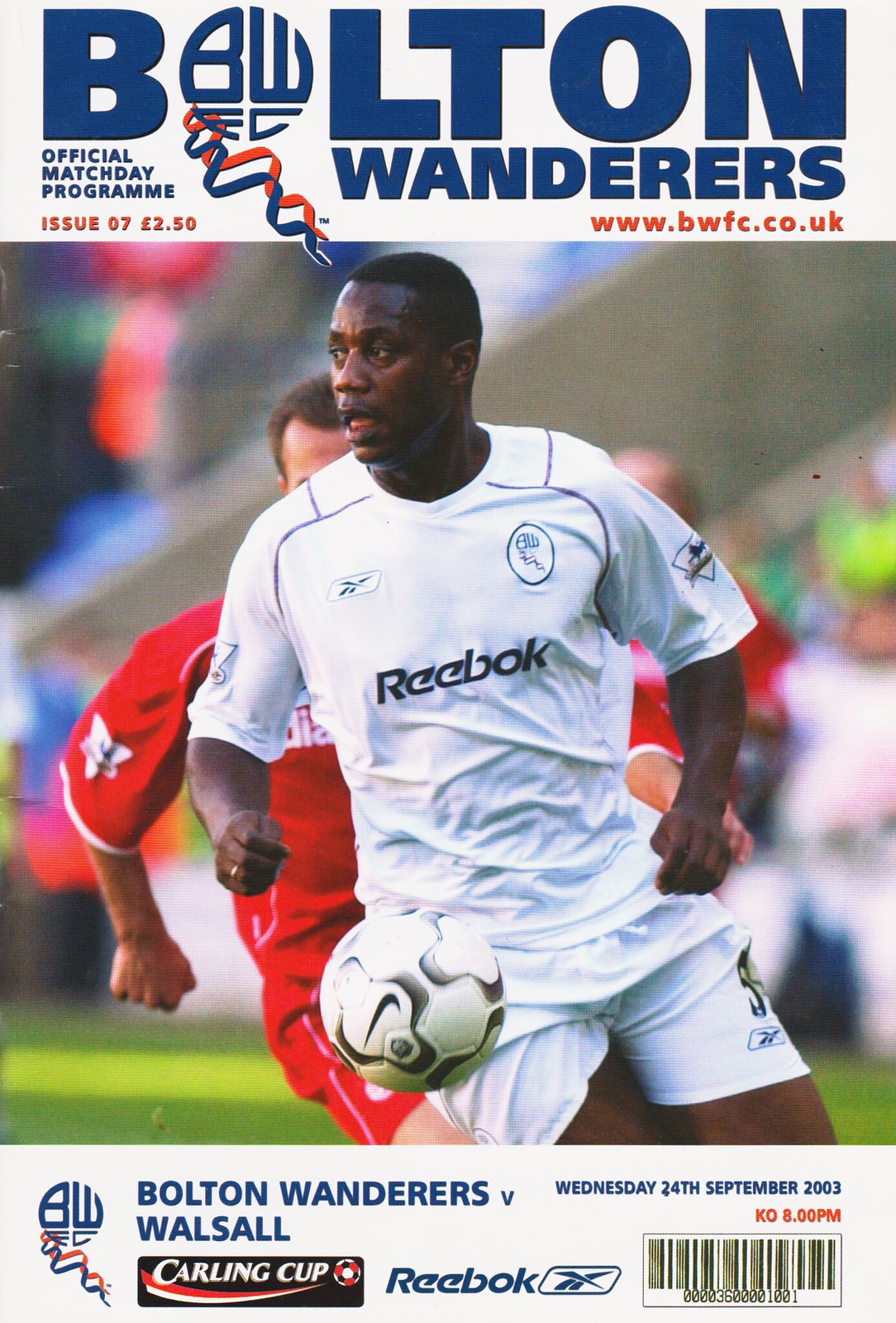The cover of the magazine is for the Official Match Day Program of the British football club, Bolton Wanderers. The program, which is issue number seven, is priced at two and a half pounds and is dated Wednesday, September 24, 2003, with a kickoff time at 8 p.m. Prominently displayed at the top in bold blue text is the name of the club, "Bolton Wanderers," followed by the title "Official Match Day Program." Below, the text indicates the match details, "Bolton Wanderers vs. Walsall," also in blue.

The central image on the cover features an African-British football player from the Bolton Wanderers. He is dressed in a complete white kit - white jersey, white shorts, and white socks - with the ball positioned right in front of him. Behind him, a player dressed in red, presumably from the opposing team, Walsall, is in active pursuit. The player's jersey prominently displays the sponsor, Reebok, and the overall sponsorship for the game includes BWEC, the Carlin Cup, and Reebok. Additional details include the selling price and a barcode placed in the lower right-hand side. 

Overall, the cover is a dynamic and detailed representation of the match day event, designed to engage fans with essential match information and visually compelling imagery.